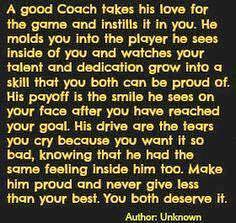The image presents an inspirational quote against a black background, adorned with yellow text. The passage, centered on the image, eloquently reads: "A good coach takes his love for the game and instills it in you. He molds you into the player he sees inside of you and watches your talent and dedication grow into a skill that you both can be proud of. His payoff is the smile he sees on your face after you have reached your goal. His drive are the tears you cry because you want it so bad, knowing that he had the same feeling inside him too. Make him proud and never give less than your best. You both deserve it." At the bottom, in a slightly different and brighter yellow font, it states: "Author unknown." The text occupies nearly the entire image, emphasizing the powerful message.